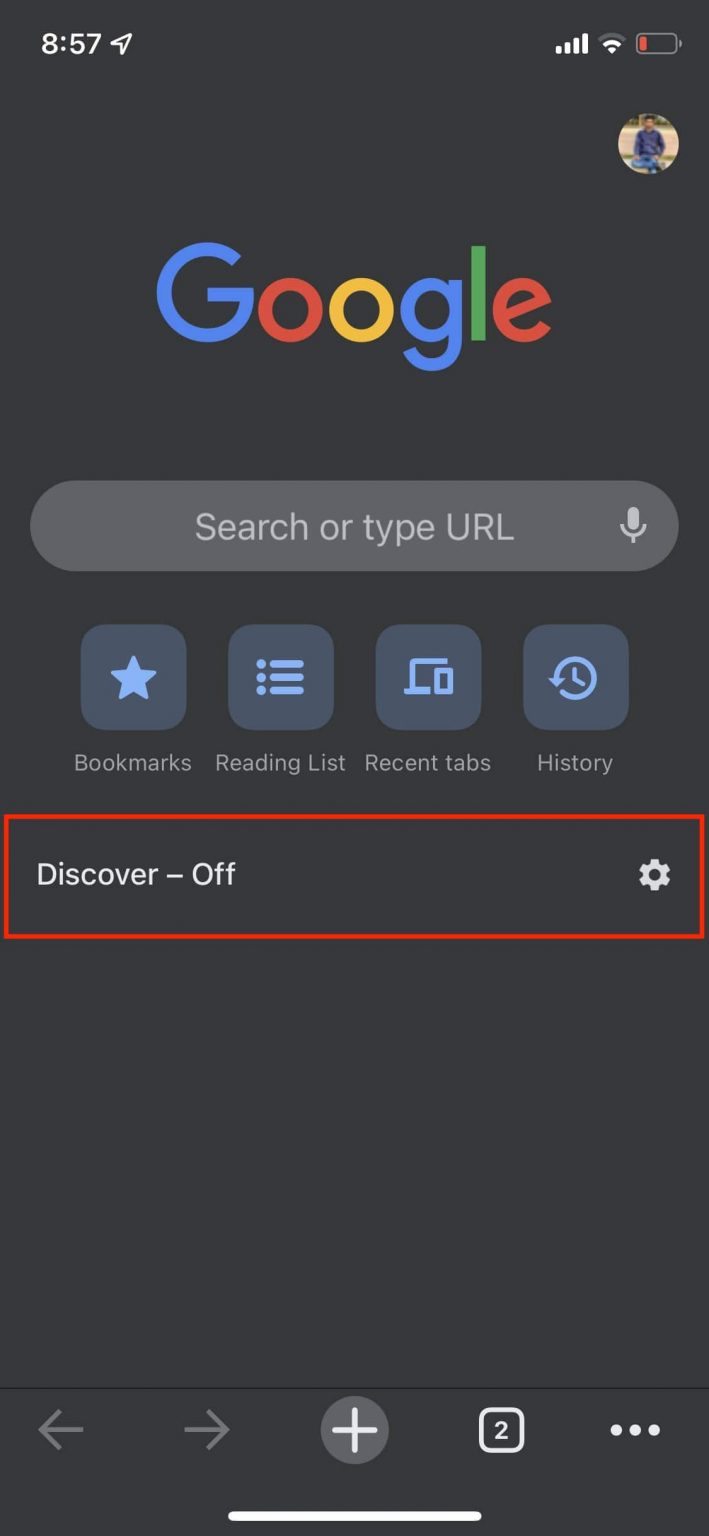A screenshot of a smartphone displaying the Google homepage. The top left-hand corner shows the time as 8:57 with a small arrow icon beside it. In the top right-hand corner, there are cellular data bars, a Wi-Fi signal icon, and a battery life indicator showing low battery in red. Adjacent to these icons is a small profile picture of a man sitting with his legs crossed, wearing purple and blue attire.

The main portion of the screen features the Google logo in blue, red, orange, and green against a completely black background. Below the logo is a search bar with the text "Search or type URL" inside it, accompanied by a small microphone icon on the right side.

Under the search bar are four rectangular boxes with icons:
1. Bookmarks - represented by a star.
2. Reading List - featuring several horizontal lines.
3. Recent Tabs - displayed with three stacked lines.
4. History - shown with a clock icon and an arrow.

Further down, there is a section labeled "Discover - off" accompanied by a white cogwheel icon, all within a rectangular red outline. 

At the very bottom of the screen, there are several navigation icons, including one resembling a phone, a plus button, a "2", and an icon with three dots and two different arrows.